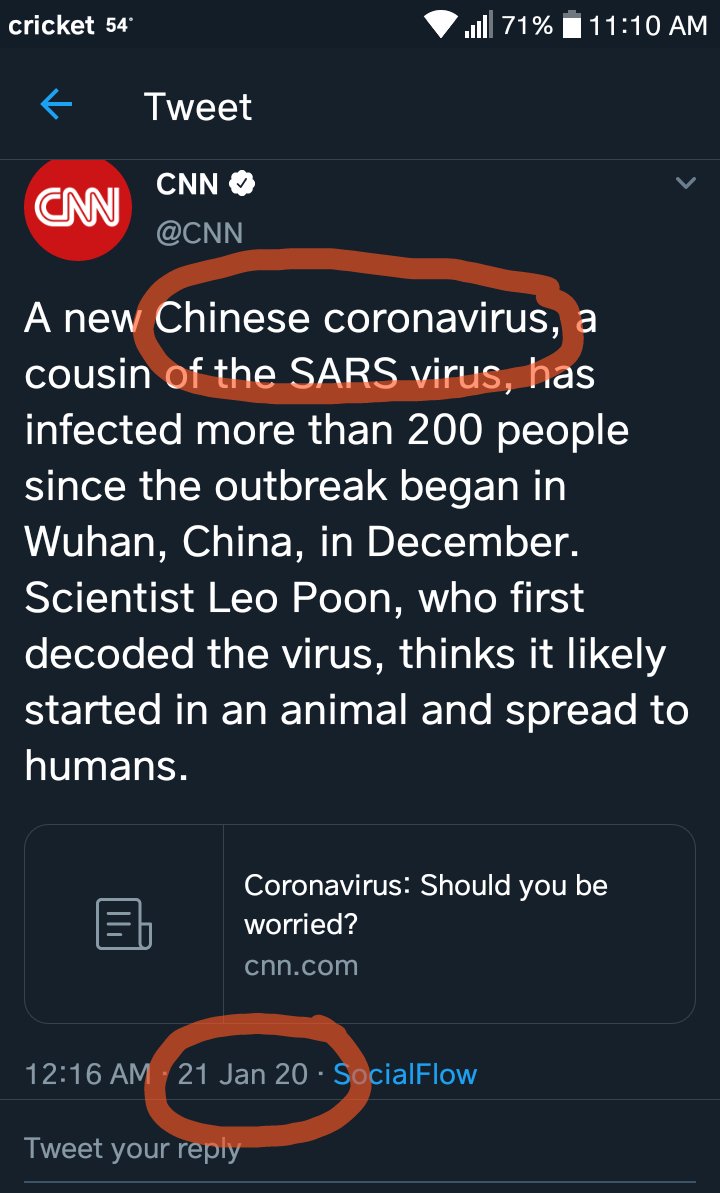This screenshot captures a smartphone display featuring a Twitter post from CNN. The background gradient transitions subtly from very dark gray at the top to a slightly lighter dark gray at the bottom. 

At the upper left corner, in white font, it shows "Cricut 5.4." The upper right corner displays the time "11:10 AM" in white font, alongside icons indicating a 71% battery charge, wireless connection, and WiFi status. 

Below these details, the screen displays "Tweet" in white font, confirming this is from Twitter before its rebranding to X. On the left side, there's a blue arrow pointing to the left, located below the CNN logo—a red circle with the stylized capital letters "C-N-N" in white. Next to the logo is "CNN" against the dark gray background, along with a verification checkmark, and the handle "@CNN."

The tweet's content reads: "A new Chinese coronavirus, a cousin of the SARS virus, has infected more than 200 people since the outbreak began in Wuhan, China, in December. Scientist Leon Poon, who first decoded the virus, thinks it likely started in an animal and spread to humans." Beneath this message is a link labeled, "coronavirus, should you be worried?" directing to an article on CNN.com. 

At the very bottom, the date "12:16 AM - Jan 21, 2020" is circled in red, indicating when this tweet was posted.